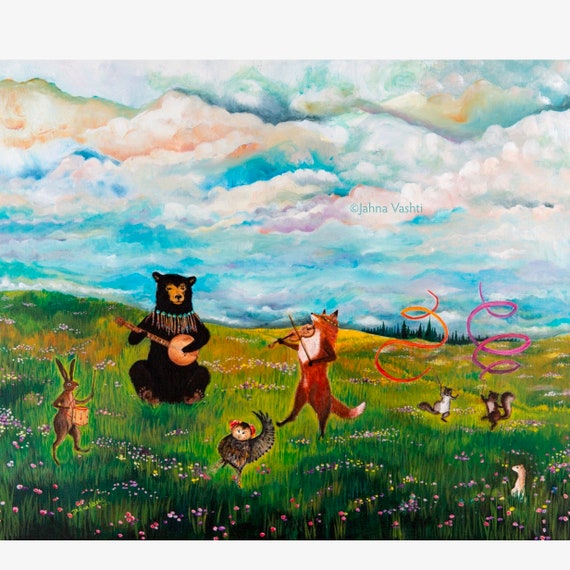This watercolor painting by Jana Vashti depicts a whimsical, daytime scene set in a vibrant, hilly meadow. The sky is a mesmerizing blend of fluffy white clouds with multicolored highlights in shades of blue, purple, pink, and orange, though it is clearly not a sunset. The lush grass in the field features two distinct shades of green, along with tall patches dotted with small pink, yellow, and purple flowers.

In this fantastical landscape, a group of anthropomorphized animals are engaged in a lively gathering. In the background, two squirrels—the male twirling a purple ribbon and the female a red one—dance with twirling streamers. The foreground showcases a charming animal band: a bear adorned with a tassel-like necklace plays the banjo, a fox with a white chest and red fur stands on its hind legs playing the violin, a rabbit on its hind legs beats a drum, and an owl wearing red headphones raises an arm as if dancing. In the bottom right corner, a small burrowing mammal, likely a meerkat, peeks out to watch the delightful scene unfold.